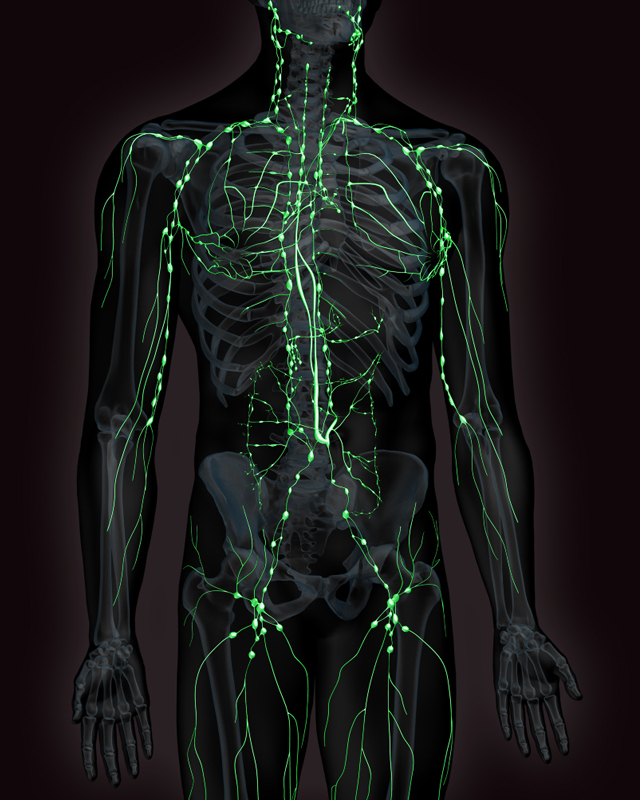This vertically aligned rectangular image depicts a computer-generated representation of a human body against a solid black background. The visible section starts just below the nose and extends down to just above the knees. The body is colored in dark gray with detailed light gray shading that indicates the skeletal frame. Prominently featured throughout the body are neon green lines and spots, likely representing veins or nerve pathways. These green lines run from the neck and chin, down across the chest, heart, arms, shoulders, and legs. Additionally, the green elements appear dendritic, branching out in various directions. The palms of the hands face outward, contrasting the stark black background that fades to a light gray aura surrounding the entire figure, enhancing the visibility of the green-lined pathways.